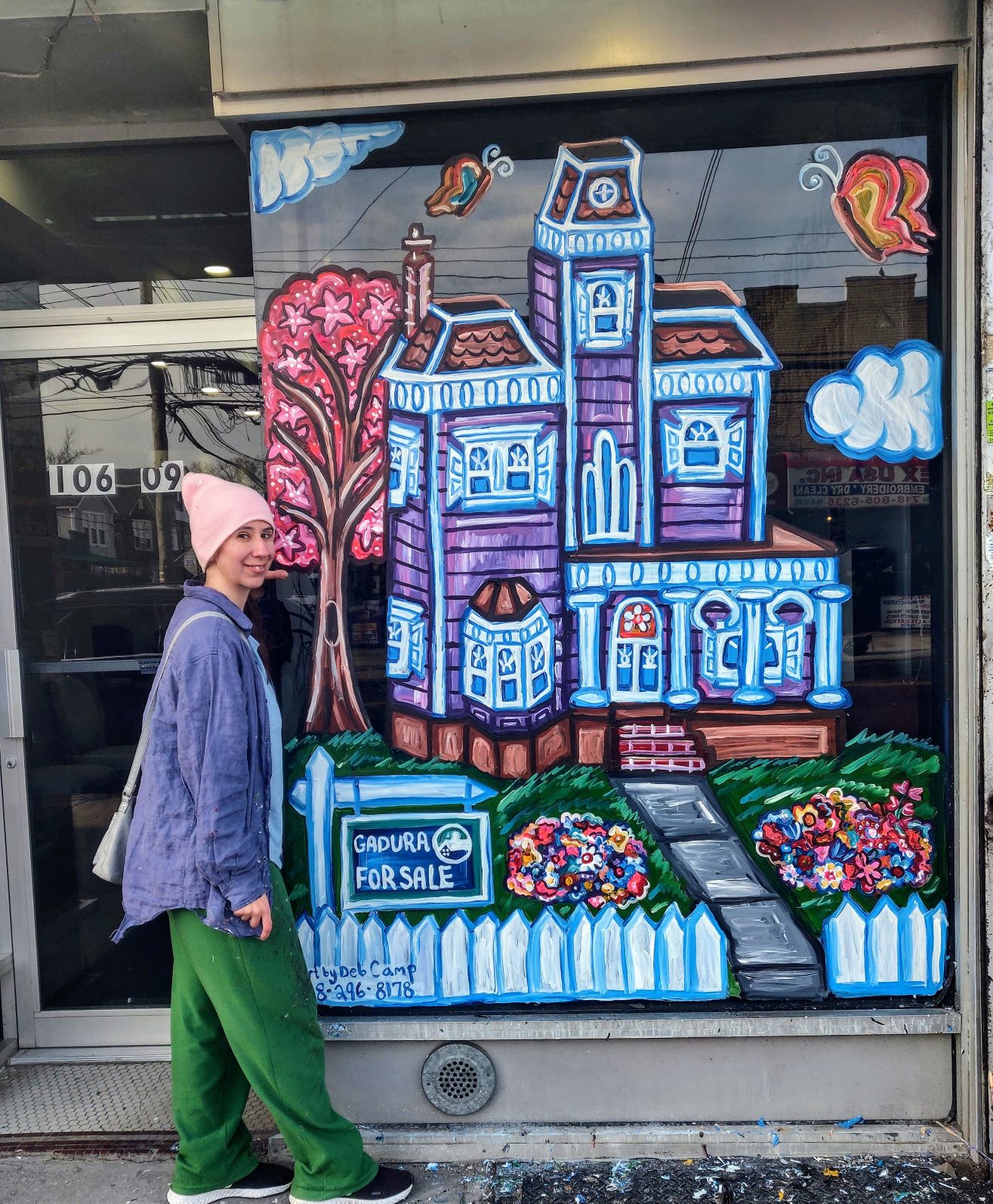This detailed color photograph features a woman standing outside next to a storefront window, which showcases an elaborate painting on the glass. The window art depicts a charming, old Victorian-style house painted in purple with blue trim, a brown roof, chimneys, and a central tower. The house has white-framed windows, a columned porch, and a red brick stairway leading to a gray walkway lined with a white picket fence. In front of the house, a white on blue sign states "Ghidorah for sale," and the artwork is signed DCAMP with the number 296-8176 below. Above the house, there are white clouds, butterflies, and what appear to be snails. Accompanying the house is a pink tree adorned with pink flowers. The storefront window is labeled with black text on white stickers displaying the number 10609. The woman, who is looking towards the camera, is wearing a pink knit hat, a purple long-sleeve shirt with a pink hoodie, green pants, black and white shoes, and a white purse. She stands to the left of the window, near the entryway to the store.